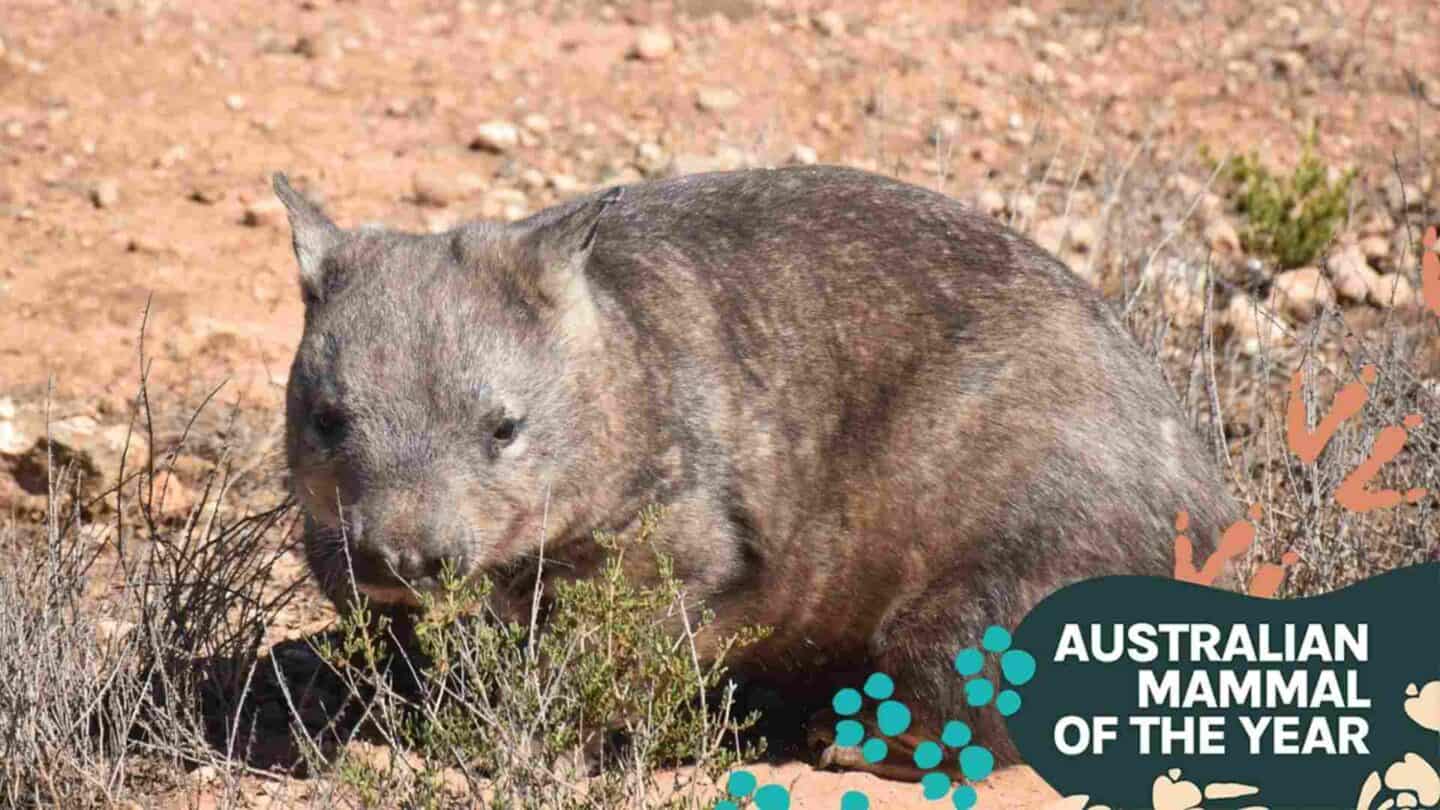This image features a small, brown animal with thin fur and noticeable pink parts, including a prominent nose and upright ears. The creature is situated on a sandy ground interspersed with grasses and various plants – some leafy and others barren. In the bottom right corner, there is a text overlay that reads "Australian Mammal of the Year," accompanied by blue-drawn footsteps on its left side. The background shows a mix of sand and rocks, completing the scene. The animal, though not explicitly identified, appears to be an unusual and intriguing example of Australian wildlife, potentially even a baby kangaroo or another peculiar mammal, adding to its enigmatic charm.